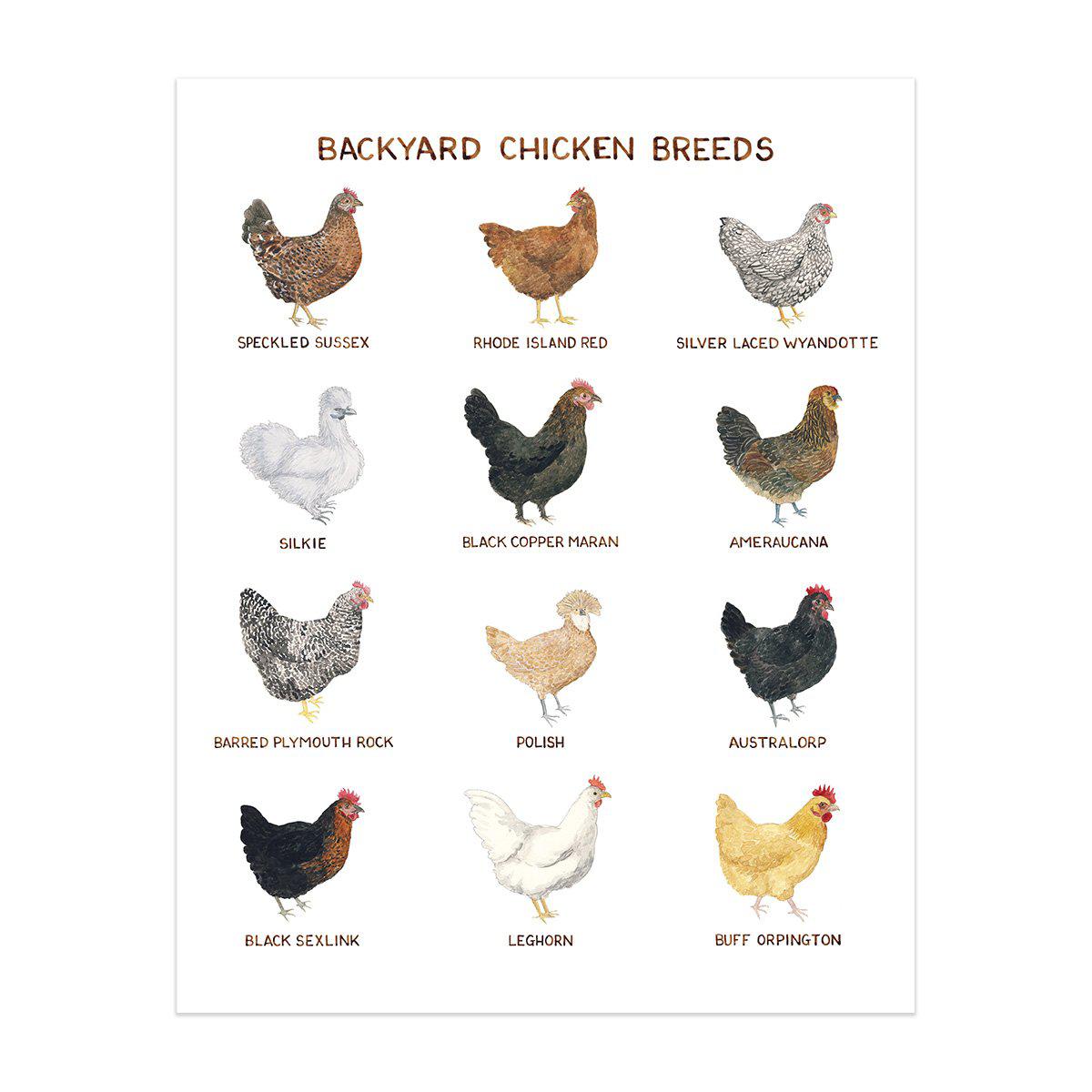The poster titled "Backyard Chicken Breeds," displayed on a white background with brown text, showcases a variety of chicken breeds. It features 12 chickens, each depicted in a side-view illustration looking to the right, organized into four rows and three columns. Starting from the top, the breeds listed are as follows: 

1. Speckled Sussex, a brown chicken;
2. Rhode Island Red, a reddish-brown chicken;
3. Silver-Laced Wyandotte, a black and white chicken with red accents;
4. Silky, an all-white chicken;
5. Black Copper Maran, a black chicken with red plumes;
6. Americana, which showcases a mix of light and dark brown with a red head;
7. Barred Plymouth Rock, identified by its black and white specks and red head;
8. Polish, a brown chicken with a distinctive tuft of feathers on its head;
9. Australorp, jet black with red accents;
10. Black Sexlink, mainly black with a brown breast and red head;
11. Leghorn, white with a red head;
12. Buff Orpington, tan with a red head.

The visual arrangement and descriptive details effectively highlight the diverse characteristics of each breed.